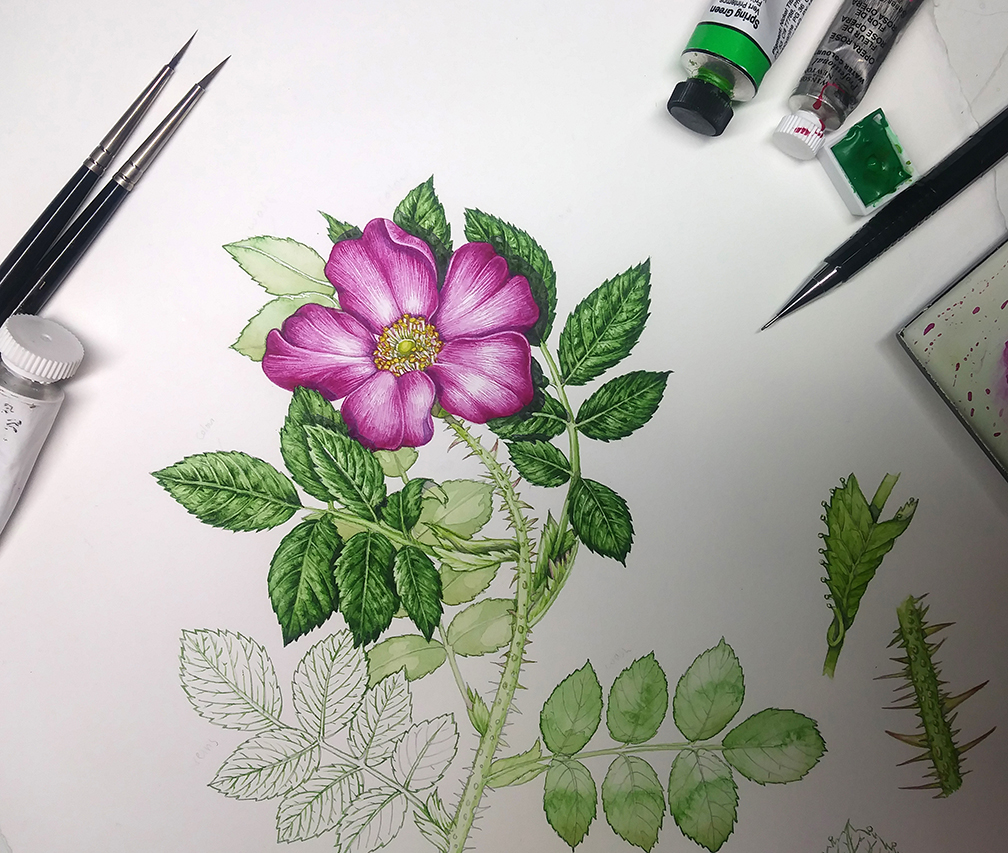The image captures an artist's workspace featuring an incomplete painting of a highly detailed purple flower with a yellow and white center, set against a white background. The painting prominently displays an intricate arrangement of green leaves and vines extending downward and off the page, with some leaves left unpainted, indicating the piece’s unfinished state. To the left of the painting are two fine-tipped paintbrushes, a silver tube of paint with a white lid, and an open barrel containing green paint. On the right side, additional art supplies are visible, including another pair of paint tubes—one green with a black cap, the other clear showing black ink—and a small pen likely used for sketching. Below these tools is a tiny square container holding green paint. The artist's meticulous preliminary sketches for the vines and stalks are also evident on the right side, ready to be brought to life on the canvas. The overall scene is a vivid testament to the artist's detailed process and the evolving nature of their work.